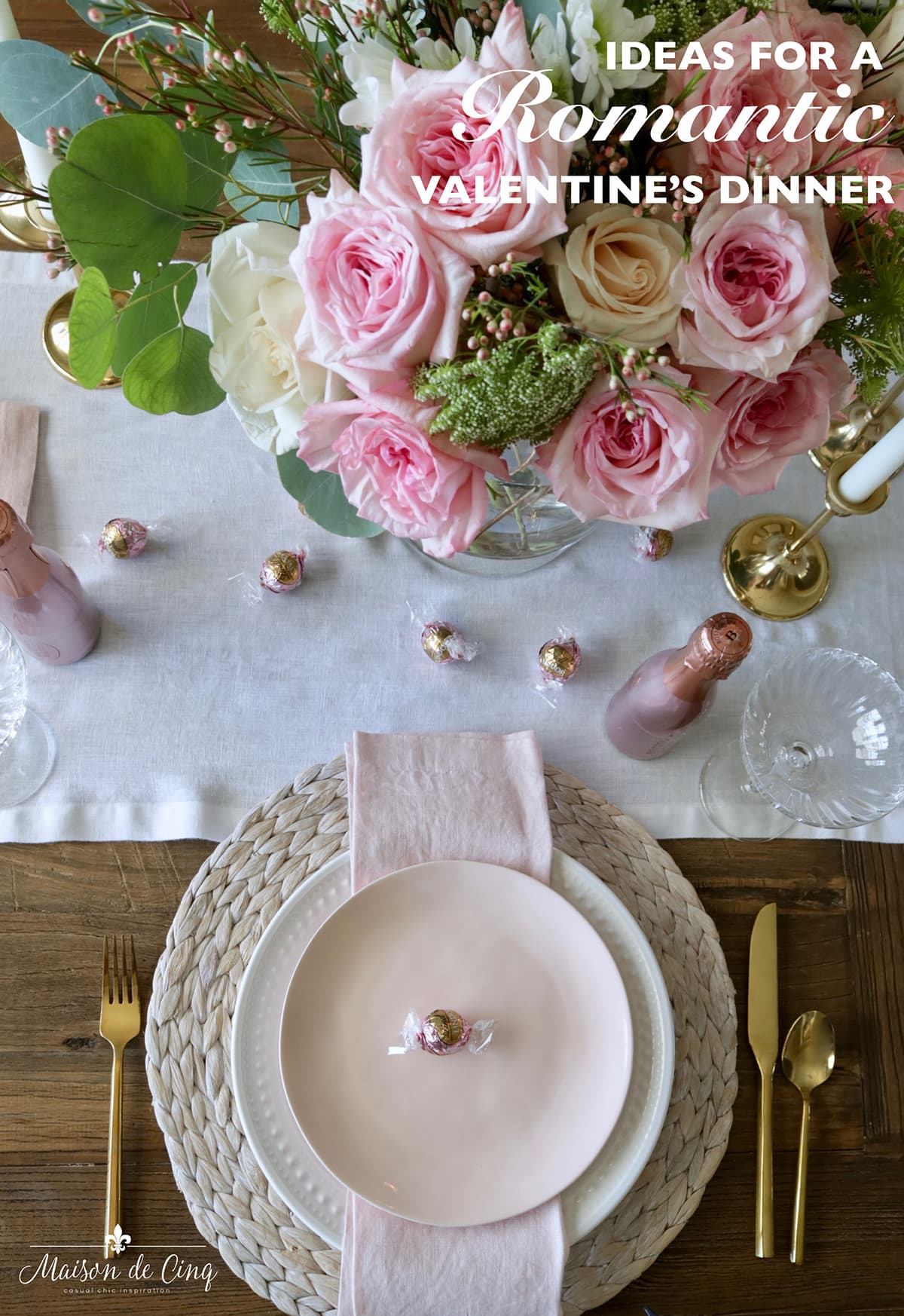The image is a detailed portrayal of a beautifully arranged Valentine's dinner idea, highlighted with a white text in the top right corner stating, "Ideas for Romantic Valentine's Dinner." The photograph is a top-down view showcasing a table set with a white linen tablecloth, adorned with a bouquet of pink and white roses nestled in a vase with greenery. Gold candle holders with white candlesticks are elegantly placed on the table, accompanied by clear champagne glasses and small pinkish champagne bottles. There are pieces of candy wrapped in gold paper and cellophane distributed across the table. The table setting includes a white plate atop a white wicker circular table mat, with gold silverware placed on either side. An off-white, slightly pinkish plate with an additional piece of candy lies across a neatly folded napkin. In the bottom left, the text reads "Mason de Sing," possibly indicating the hosting website, while the author's name, "Marsandi Ong," is noted beneath the tableware setup. The scene is set on a rich, brown wooden table, enhancing the romantic and elegant ambiance.